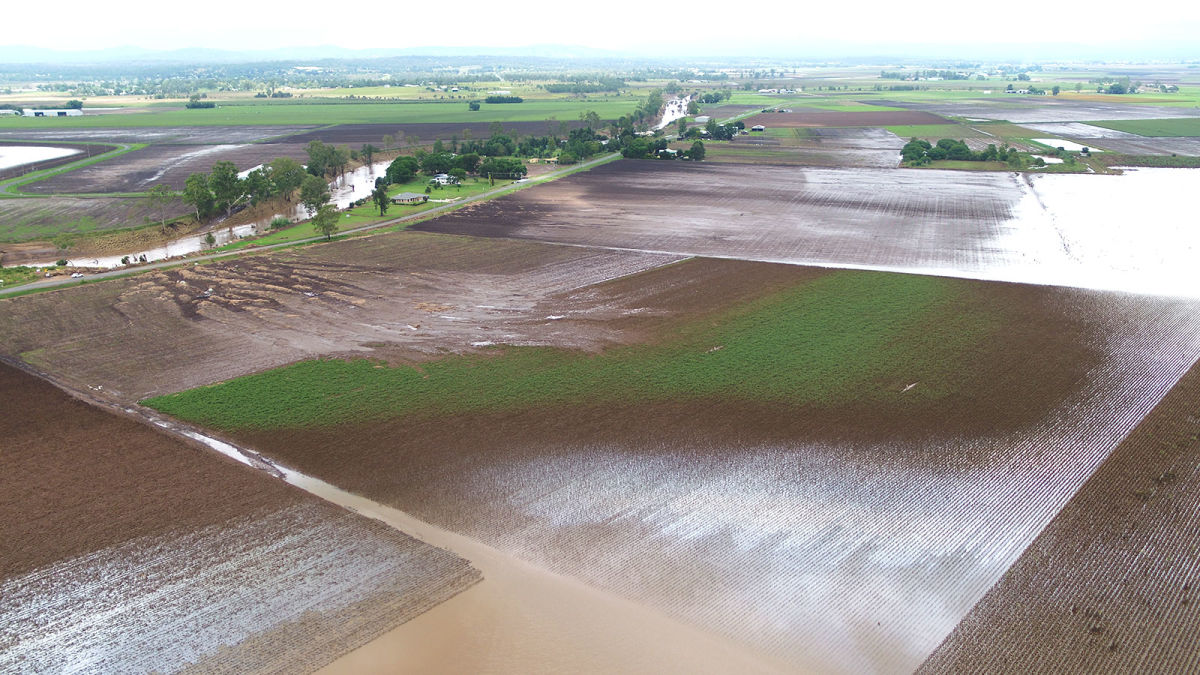The image captures a meticulously organized farmland scene viewed from above, bathed in natural daylight. Dominating the foreground are large, square-shaped plots of vibrant green fields interspersed with patches of brown and muddy soil, indicating recent rainfall. Flooded canals and water patches are visible, suggesting effective irrigation or the aftermath of a substantial downpour. A narrow, old country road weaves through the landscape, bordered by these geometric fields. Surrounding this central farmland are hints of rural habitation, with small clusters of houses and buildings. In the background, a vivid blue sky merges with a low-lying mountain range, adding depth to the serene, pastoral setting. The overall composition of the image highlights the well-maintained nature of the farmland, reflecting a blend of lush greenery and productive soil, framed by distant natural and architectural elements.